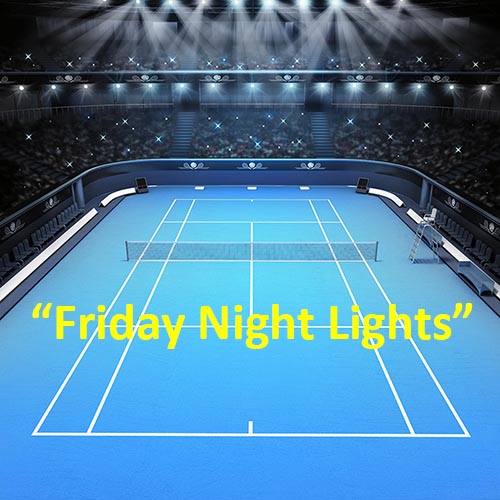The image captures a detailed view of a tennis arena from an elevated perspective, looking down at a pristine blue tennis court framed by crisp white lines. The net stretches horizontally across the court, with the umpire's chair positioned on the right side. The court is bordered by a sleek, see-through blue acrylic wall, legible by white and black stripes at the base. Prominently displayed on the court is a motivational yellow text, "Friday Night Lights," emphasizing the event's dynamic atmosphere.

The arena is bustling with an audience spread across multiple tiers, their presence illuminated by numerous white lights and cell phone screens, contributing to the lively ambiance. Above the court, powerful stadium lights cast a bright glow, enhancing visibility. In the areas where judges, players, and ball boys typically position themselves, the seats are currently vacant, suggesting a moment of intermission or pre-game setup. The overall scene is a blend of vibrant activity and meticulous planning, capturing the anticipation and excitement unique to a live sports event under the lights.